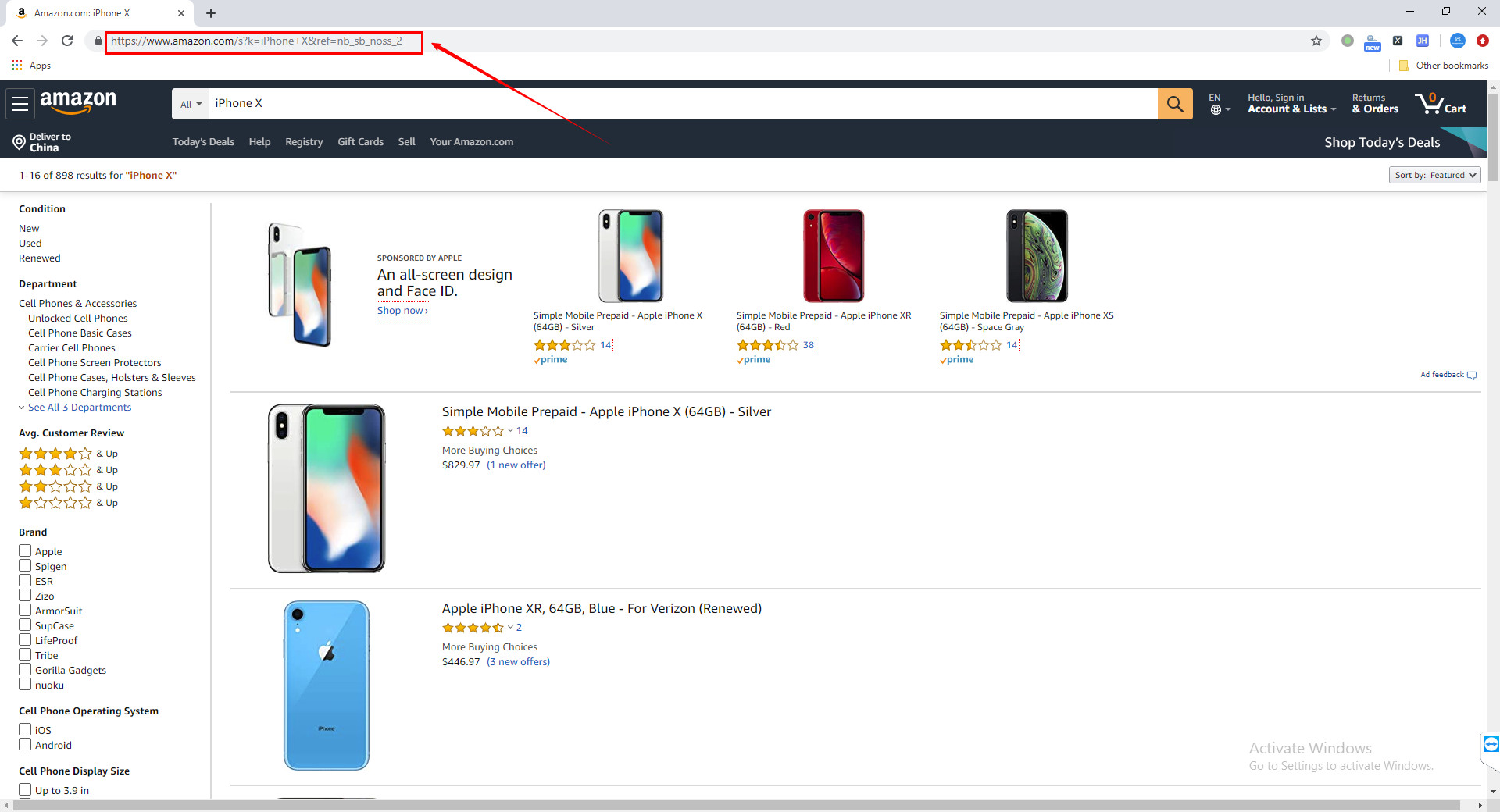The image captures a detailed screenshot of an Amazon search results page for "iPhone X." At the top of the page, there's a prominently featured sponsored listing highlighting an iPhone X with an all-screen design and Face ID, available in various color options. Below the sponsored listing, the first non-ad result displays a Simple Mobile prepaid iPhone X in silver, rated 3 stars out of 5 based on 14 reviews. Further down, another listing showcases a renewed iPhone XR with 64GB storage in blue, compatible with Verizon, boasting a rating of approximately 4.5 stars from 2 reviews. The prices are somewhat challenging to decipher, but the renewed iPhone XR appears to be priced around $450, while the new iPhone X is listed at roughly $830. An annotated arrow is suggested to be added, pointing to the address bar which reads "Amazon.com," followed by some illegible characters. The address bar detail is marked as notable despite its unreadability.